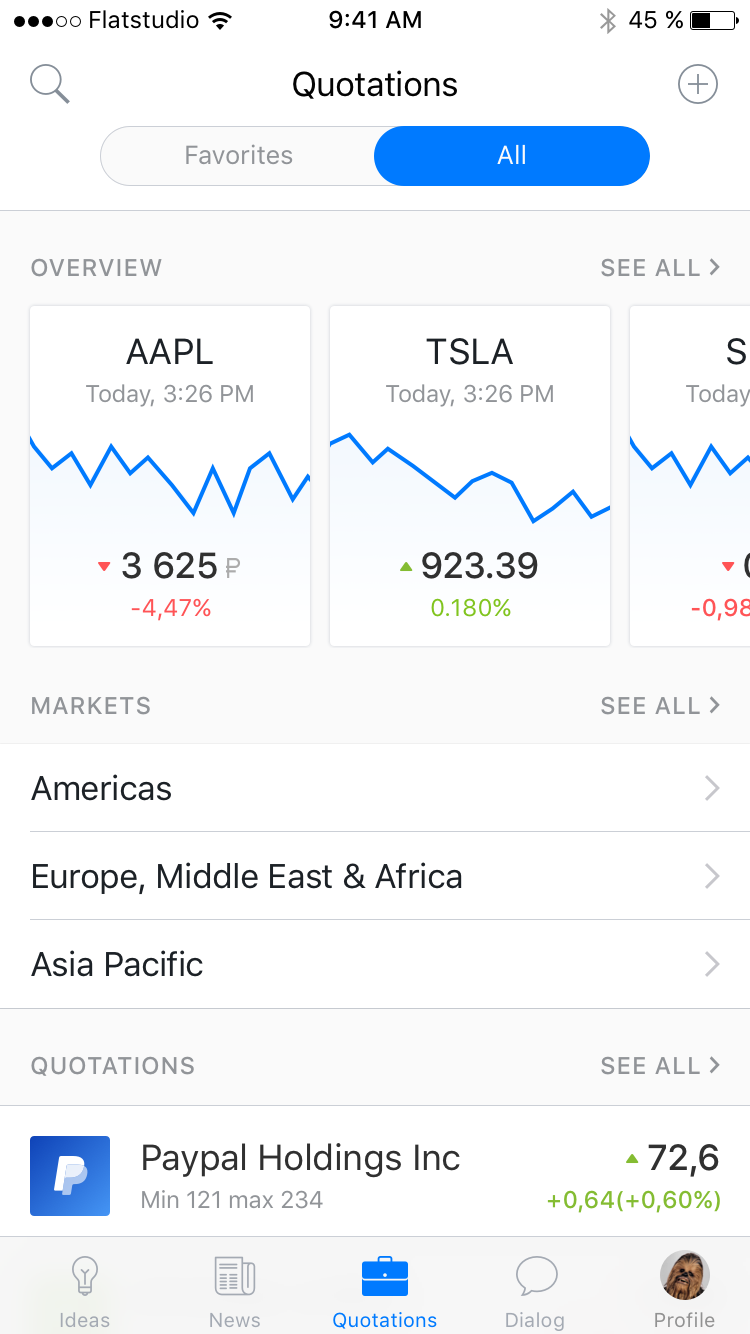The top portion of the image includes three black circles and two white circles, indicating different statuses or metrics. It also displays "Flat Studio" prominently, alongside several status icons: a Wi-Fi icon, a 9:41 AM timestamp, a Bluetooth icon, and a battery indicator showing 45%.

Beneath this, there is a search icon followed by the heading "Quotations." Adjacent to this is a circular icon with a plus sign inside it. There are two buttons below the heading: a gray button labeled "Favorites" and a blue button labeled "All."

Following these buttons, there are several sections. The first section reads "Overview," with an option to "See All." Below, there's graphical data organized within boxes. 

In one box, labeled "AAPL Today, 3:26 PM," a red arrow points downward, indicating a decline, with values reading "3,625" and "-4.47%." Right next to it, another box labeled "TSLA Today, 3:26 PM" shows a green arrow pointing upward, indicating an increase, with a value of "0.180%."

Additional sections include "Markets" with a "See All" option and subsections labeled "Americas," "Europe, Middle East, and Africa," "Asia Pacific," and "Quotations," also with an option to "See All."